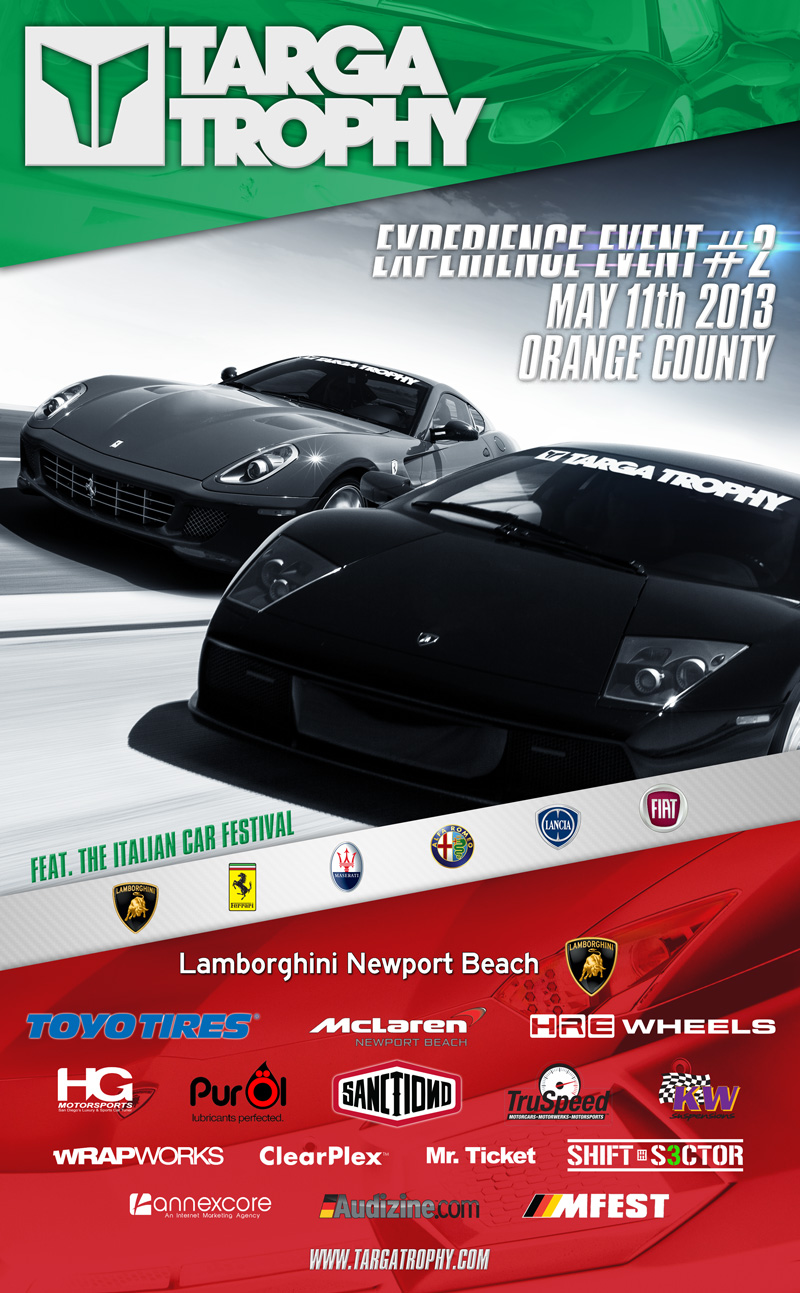This image is a detailed advertisement poster for the "Targa Trophy Experience Event Number 2," held on May 11, 2013, in Orange County. At the top left corner, the text prominently announces the event. Below this announcement, there is a photograph of two black race cars with tinted windows, both bearing the "Targa Trophy" logo across their windshields and positioned centrally within the image. The event features the "Italian Car Festival," displaying logos of prominent car brands such as Lamborghini, Porsche, Fiat, and others underneath this headline. Along the bottom of the poster, a range of sponsor logos are visible, including names like Lamborghini, Newport Beach, Toyo Tires, McLaren, HRE Wheels, Shift and Sector, Mr. Ticket, ClearPlex, Wrapworks, and several additional companies. The image incorporates a diverse color palette including red, white, black, blue, orange, yellow, green, and tan, emphasizing a vibrant and engaging visual style suitable for a promotional race event.